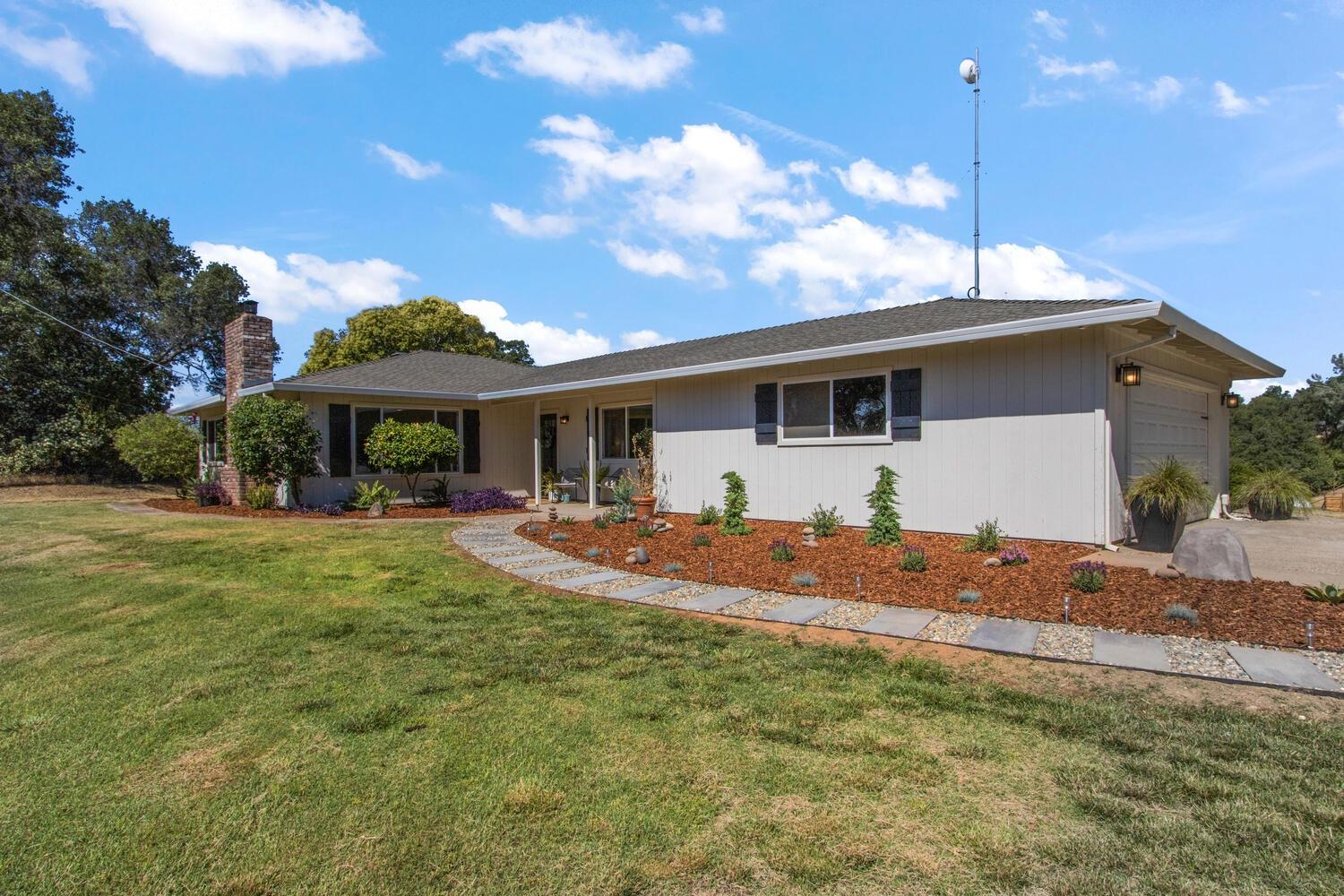This image showcases a charming ranch-style house on a bright, sunny day beneath a beautiful blue sky dotted with white, puffy clouds. The single-story white house features three slider windows with black shutters, a feature repeated across multiple observations. A distinctive stone pathway leads from the right-hand side, curving gracefully toward the front door, which is sheltered by an overhang supported by two poles. Adjacent to the front door, a light fixture is attached to the wall, illuminating the entryway.

The house is framed by a meticulously maintained green lawn on one side and a rock yard on the other, which hosts an assortment of succulents, cacti, and other shrubs. Additional plants, trees, and flowers intersperse the landscape around the property. The garage, located on the far right, is accompanied by two lantern-style lights and flanked by potted plants, adding a subtle flourish to the utilitarian space. A paved driveway extends from the garage, further enhancing the home's practicality.

Noteworthy architectural features include a chimney protruding from the rear side of the house and a tall antenna with a satellite dish perched on the roof, pointing to the left. The image exudes a warm, inviting atmosphere, capturing the essence of a picturesque American suburban home.